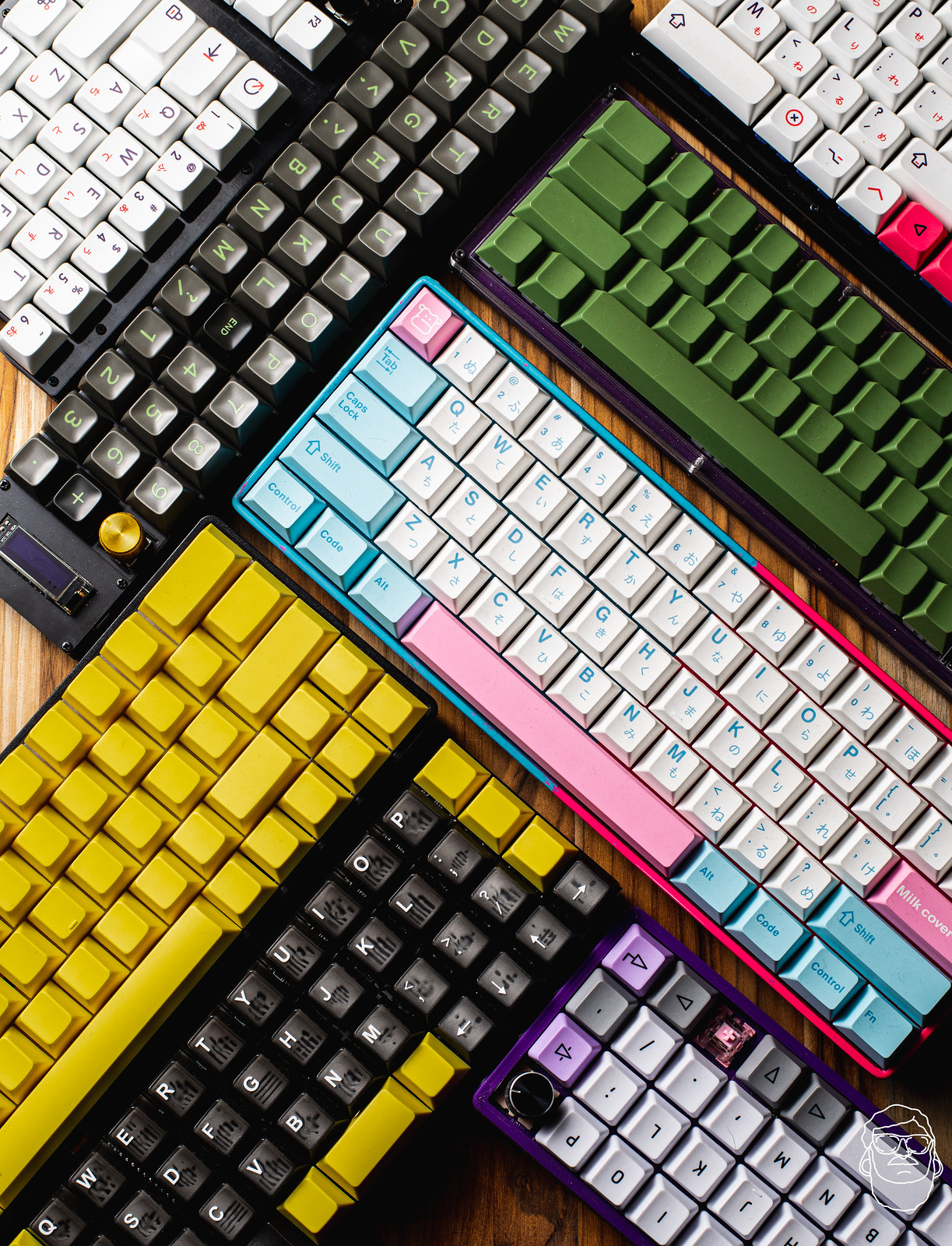This image features a visually striking arrangement of eight different mechanical keyboards displayed on a tabletop that resembles white wood with darker grain. Each keyboard showcases a unique color scheme, contributing to a geometric pattern designed for visual appeal. Among the keyboards, there is one entirely yellow keyboard with keys that have no visible numbers or letters. Another predominantly white keyboard features light blue letters, a pink space bar, escape key, and return key. Additional keyboards include an all-black one, an all-green one, and another with a purple outline. The collection also includes keyboards in brown, orange, and light blue colors. Notably, one keyboard is missing some keys. A faint watermark in the lower right corner depicts the outline of a man's face wearing sunglasses, suggesting the image might be AI-generated photorealistic art.